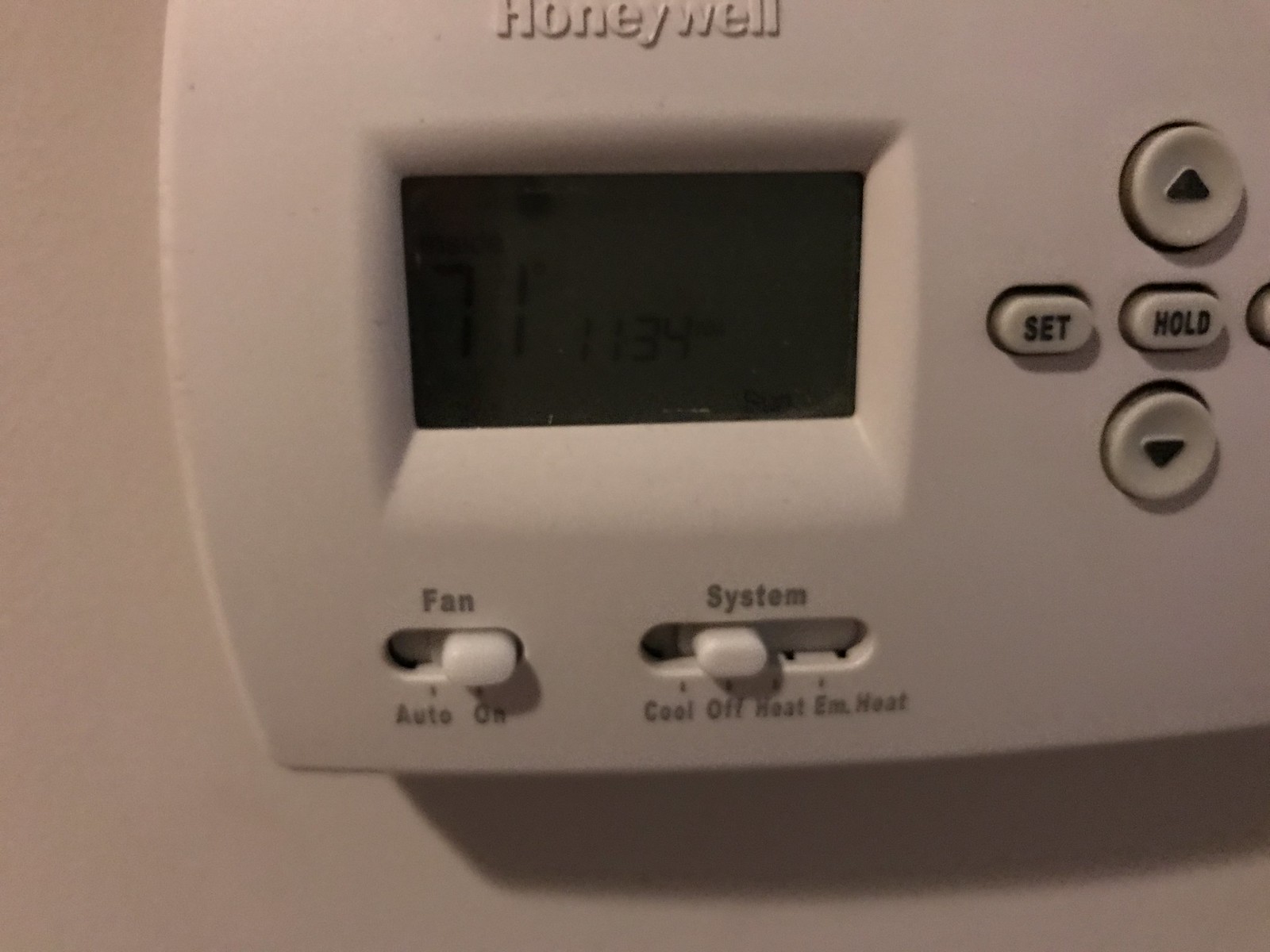The image captures a close-up of a Honeywell thermostat in a dimly-lit setting, suggesting it was taken in the evening or nighttime. The scene is illuminated by a faint, artificial light source emanating from the left side, casting soft shadows across the device and accentuating its contours. The thermostat, which is predominantly white, features a small electronic screen positioned on the left-hand side. Above the screen, the brand name "Honeywell" is embossed in raised letters. 

Beneath the screen, there are two slide switches: the first, labeled "Fan," slides from "Auto" on the left to "On" on the right. Adjacent to it, the second switch is labeled "System" and can be set to "Cool," "Off," "Heat," and "EM Heat" (Emergency Heat) in a left-to-right sequence. On the right side of the screen, there are four buttons arranged vertically. The top button is circular with an upward-pointing arrow. Below it are three oval buttons, two of which are visible and labeled "Set" and "Hold," while the third is partially obscured. At the bottom, there is another circular button featuring a downward-pointing arrow. The meticulous details of the thermostat's controls are accentuated by the interplay of light and shadow, providing depth to the image.